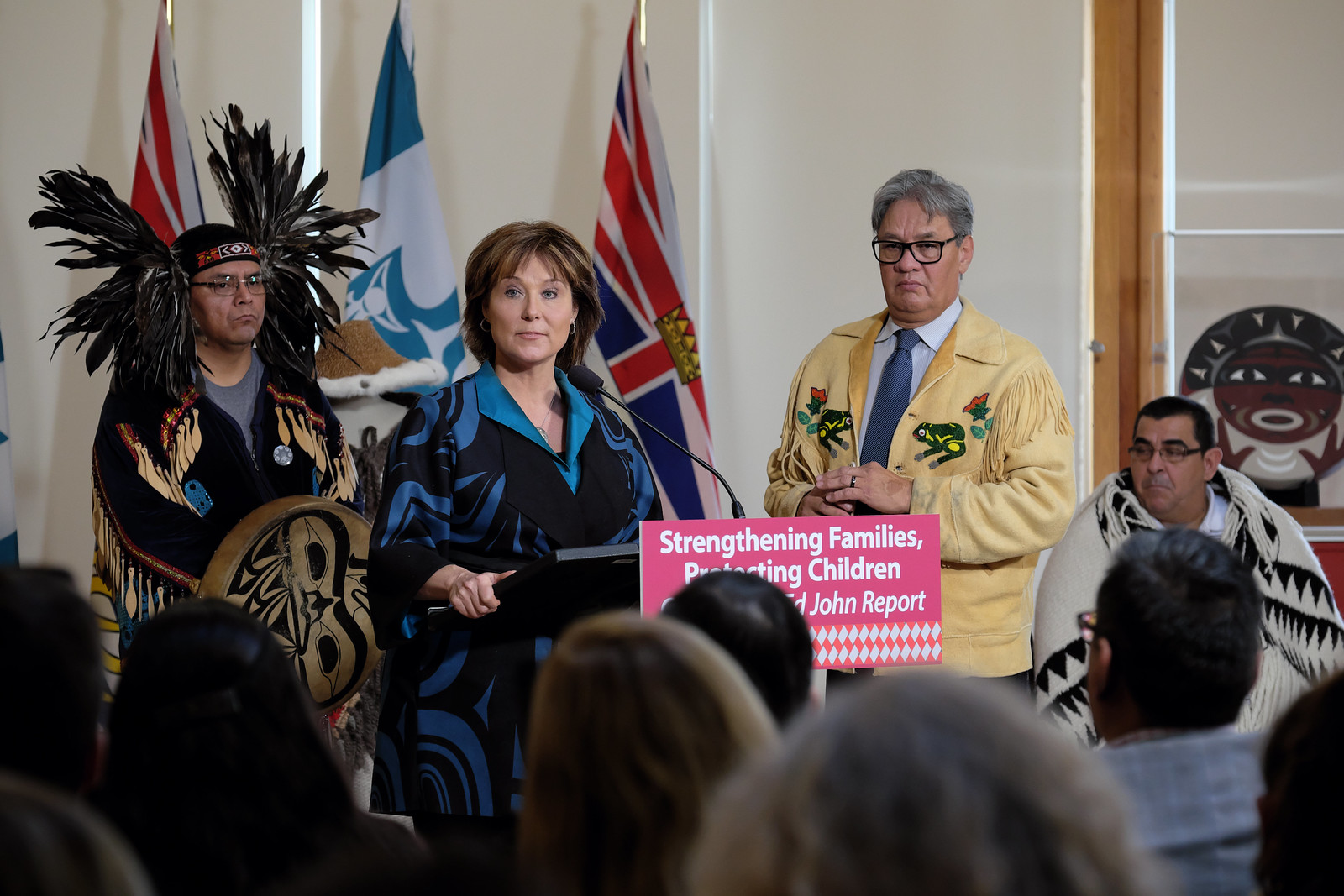At the podium, a woman stands at the microphone, dressed in a blue and black dress with short brown hair streaked with blonde highlights. Behind her, a man wearing traditional Native American attire observes attentively. To her left, another man is seen wearing a tan fringe jacket. The podium's banner prominently displays the message, "Strengthening Families, Protecting Children." The design of the lower half of the podium features a rectangular section with a pink background and two rows of white diamond patterns.